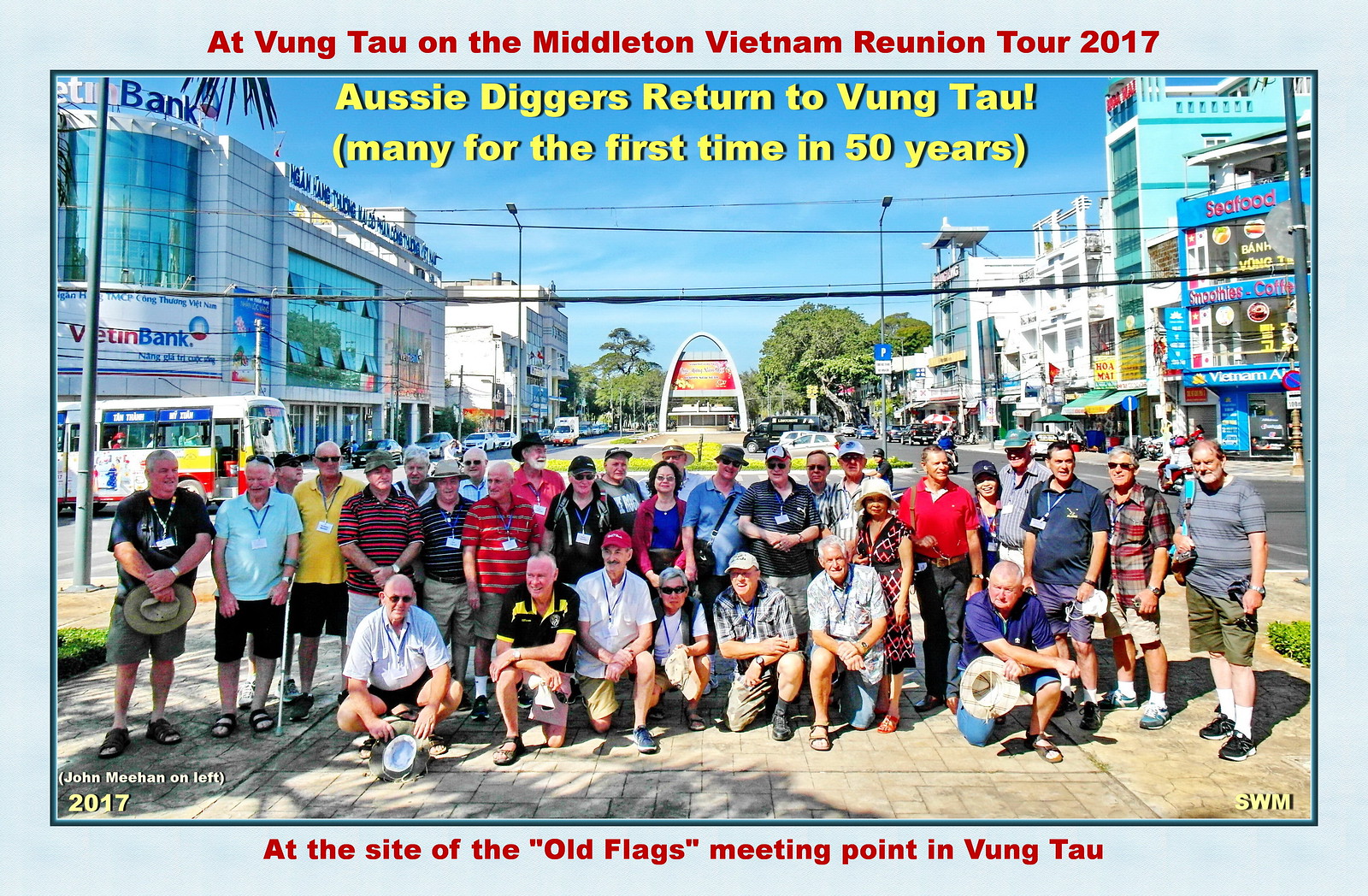This photograph, taken during the daytime on a busy city street, captures a group of mostly older individuals, likely in their 50s to 70s, gathered for the Middleton Vietnam Reunion Tour 2017 in Vung Tau. The image has a light blue border, with red letters at the top reading, "AT Vung Tau on the Middleton Vietnam Reunion Tour 2017," and text at the bottom that states, "At the Site of the Old Flags Meeting Point in Vung Tau," with additional annotations reading "John Meacham on Left 2017" and "SWM." A central line of text in yellow reads, "Aussie Diggers Return to Vung Tau, Many for the First Time in 50 Years."

The group, consisting of around 20-30 people, including three women—some of whom appear to be Asian—are diverse in attire, with men mostly dressed in shorts and a variety of colored shirts (gray, red, blue, and brown) and a few wearing red or white baseball caps. Some individuals also wear lanyards, and one man has a cane attached to his arm. The front row kneels on concrete, while the others stand behind them. They are positioned in the middle of a sidewalk, under a blue sky with visible power lines and trees in the background.

The backdrop showcases a vibrant cityscape featuring storefronts, restaurants, multicolored buildings including a teal one, and signs displaying "Seafood, Smoothies, Coffee" and "Viet Bank." A bus is seen in the left-hand corner, amidst other cars and vans, contributing to the bustling atmosphere. The detailed and commemorative nature of the photograph highlights the significance of this reunion for the veterans, many of whom are returning to Vietnam for the first time in 50 years.